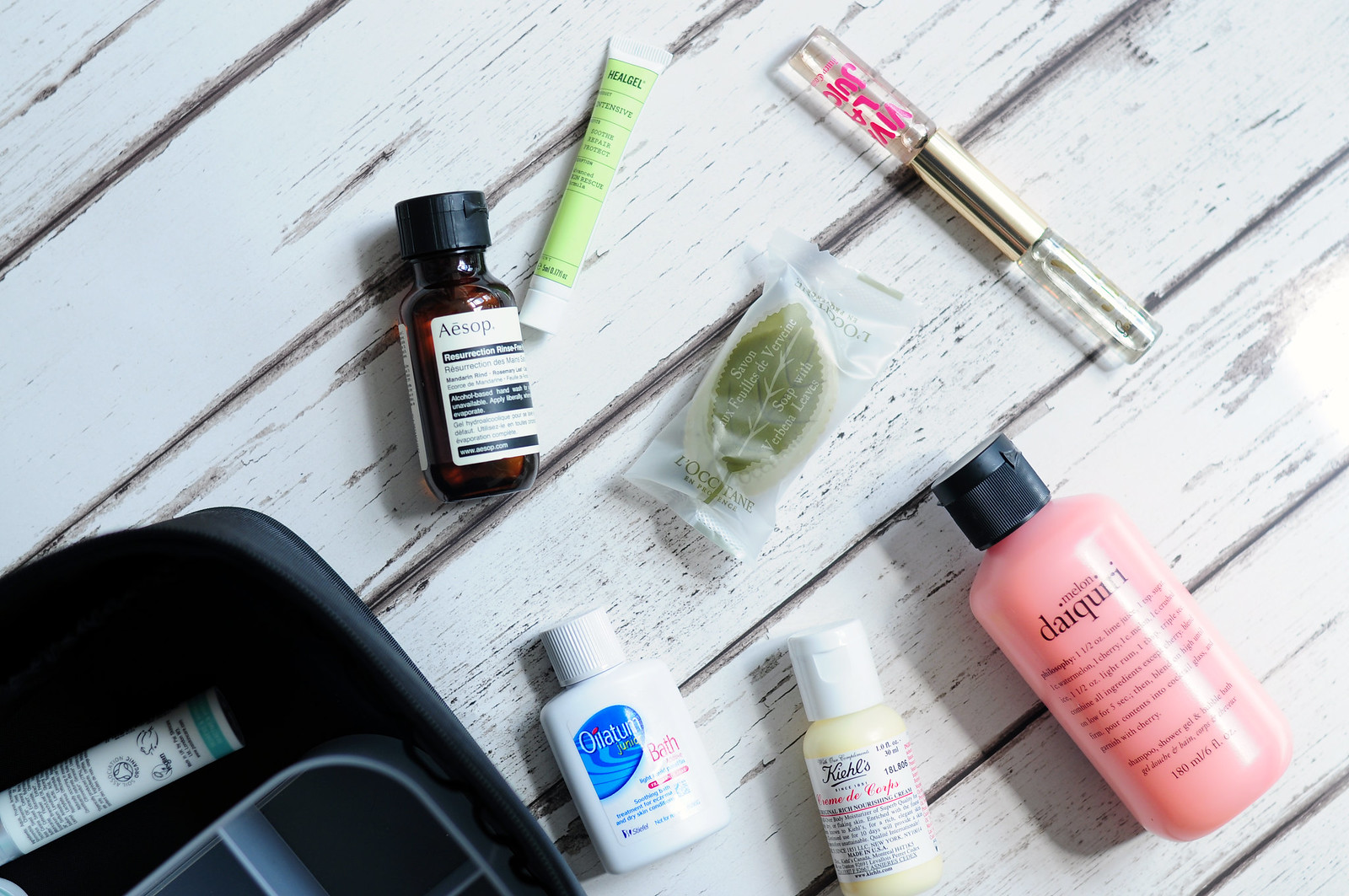This top-down product photography image features a rustic, white-painted wooden surface that's visibly worn, revealing patches of the natural wood underneath. The wooden boards run diagonally from left to right at about a 45-degree angle. Scattered atop this textured background are various makeup and skincare items, artfully arranged to maintain a pleasing, static appearance.

In the bottom left corner of the image, a small section of a bag is visible, revealing part of an additional makeup item inside—a white-colored organizer, with only about 10% of it showing. The beauty products on the surface include a brown Aesop bottle with a black screw cap, a green heel gel in a white tube, some lip gloss, soap, an orange Kiehl's bottle, a melon daiquiri bottle, and bath salts in a white bottle.

The attention to detail in this composition captures both the elegantly aged wooden background and the variety of beauty products, making for an eye-catching and well-balanced image.